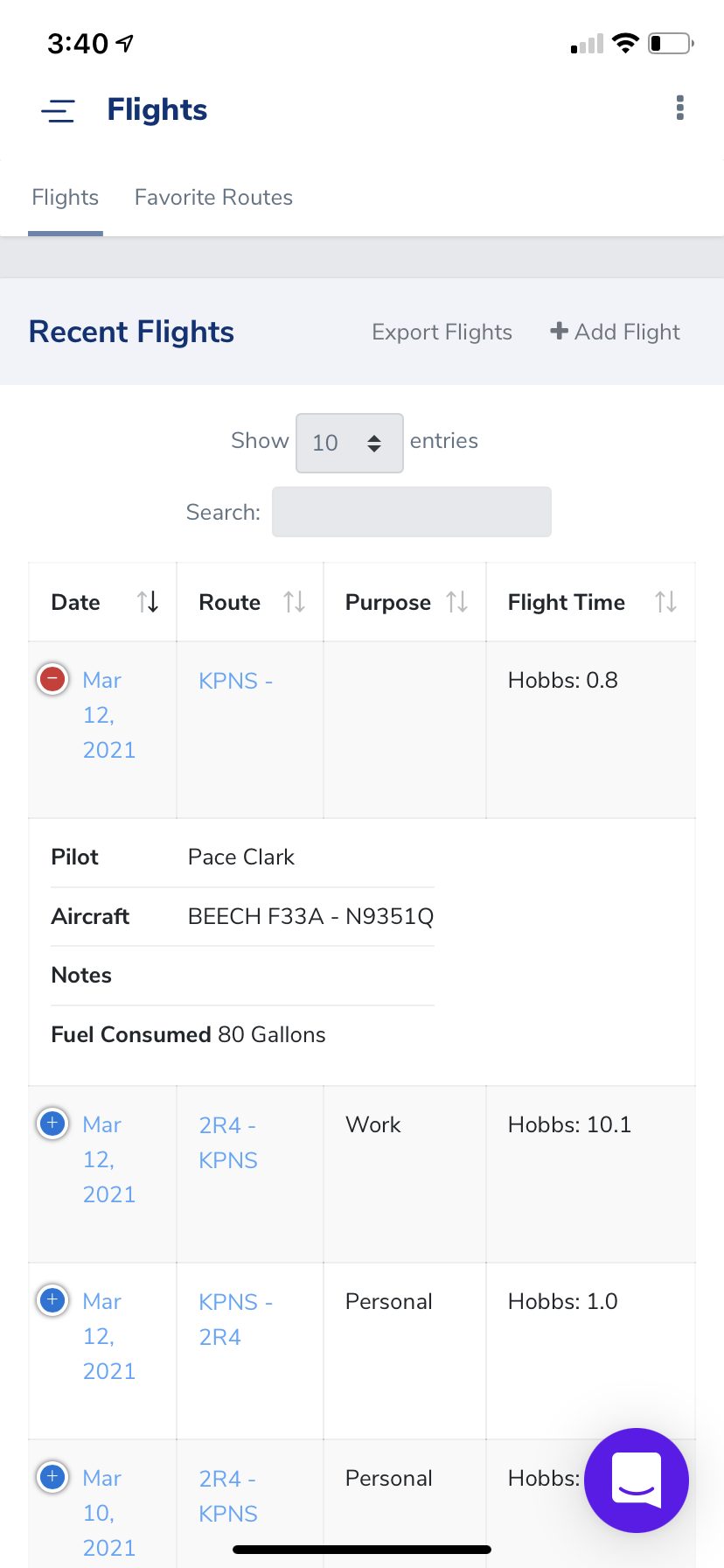The image is a screenshot of a cell phone displaying a flight information page. In the top left corner, the number "340" is shown. The top right corner features icons for cellular connection, wireless connection, and battery level. The header reads "Flights" and below it are two tabs: "Flights" and "Favorite Routes," with the "Flights" tab selected.

Under the tabs, the page section titled "Recent Flights" appears. There's a dropdown menu labeled "Show," set to display "10 Entries." Next to this is a search box, currently empty. The flight information is organized into four columns: Date, Route, Purpose, and Flight Time.

The first entry listed shows the following details:
- Date: March 12, 2021
- Route: KPNS
- Purpose: [Blank]
- Flight Time: HABS 0.8 hours

Further details are provided below this entry:
- Pilot: Pace Clark
- Aircraft: Beechcraft Bonanza, Model F33A with tail number N9351Q
- Notes: [Blank]
- Fuel Consumed: 80 Gallons

Additionally, three more flights are listed:
1. Date: March 12, 2021
   Route: 2R4 to KPNS
   Purpose: Work
   Flight Time: HABS 10.1 hours
   (A plus sign appears next to this entry)

2. Date: March 12, 2021
   Route: KPNS to 2R4
   Purpose: Personal
   Flight Time: HABS 1.0 hours

3. Date: March 10, 2021
   Route: 2R4 to KPNS
   Purpose: Personal
   Flight Time: HABS (Rest of the details are obscured by a blue or purple circle)

Due to the circle, the final entry's flight time and other details cannot be fully read.